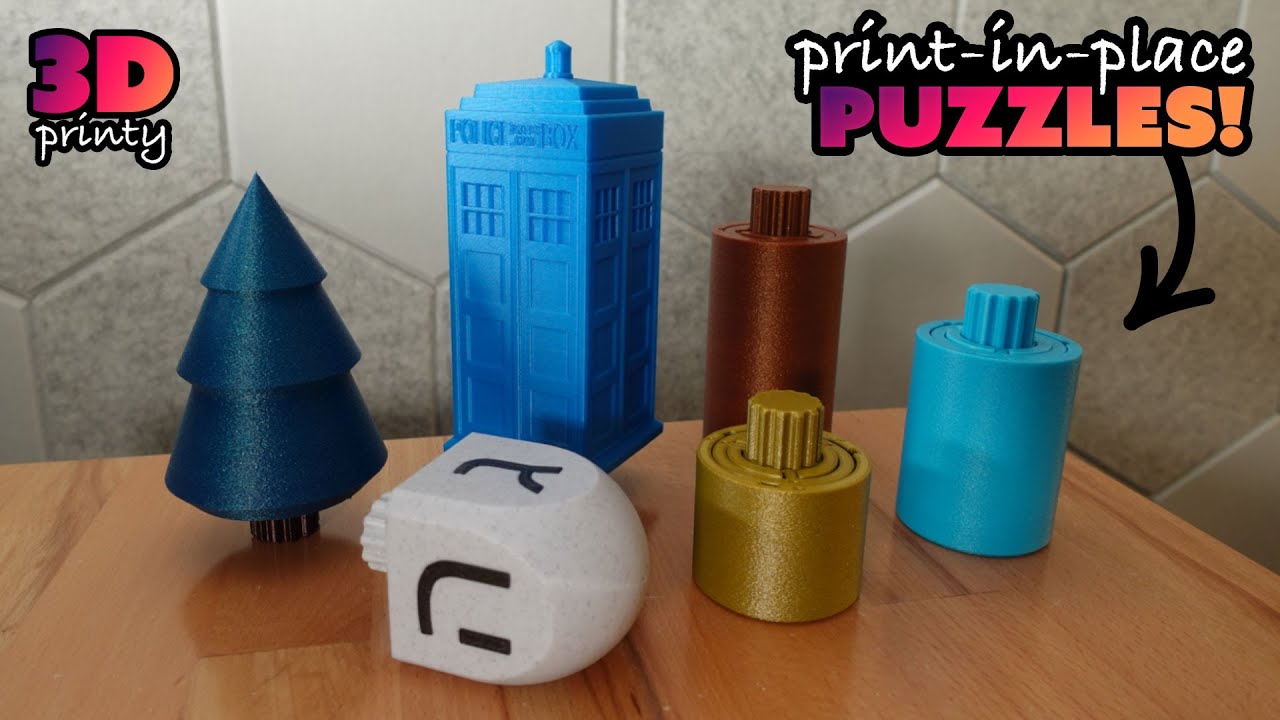The image showcases a landscape-oriented photograph featuring a wooden table set against a gray, multi-colored tiled background. On the table are six 3D-printed puzzle pieces. Dominating the scene is a dark navy blue piece shaped like a Christmas tree, and next to it, a blue one resembling a building or phone booth. In front of these, there's a white piece shaped like a dreidel with black Hebrew letters. Additionally, three cylindrical pieces resembling lotion bottles in gold, blue, and copper sit to the right. In the top left corner of the image, the text "3D Printing" is displayed, while the top right corner bears the label "Print in Place Puzzles" in colorful text with a black arrow pointing at the blue cylinder.